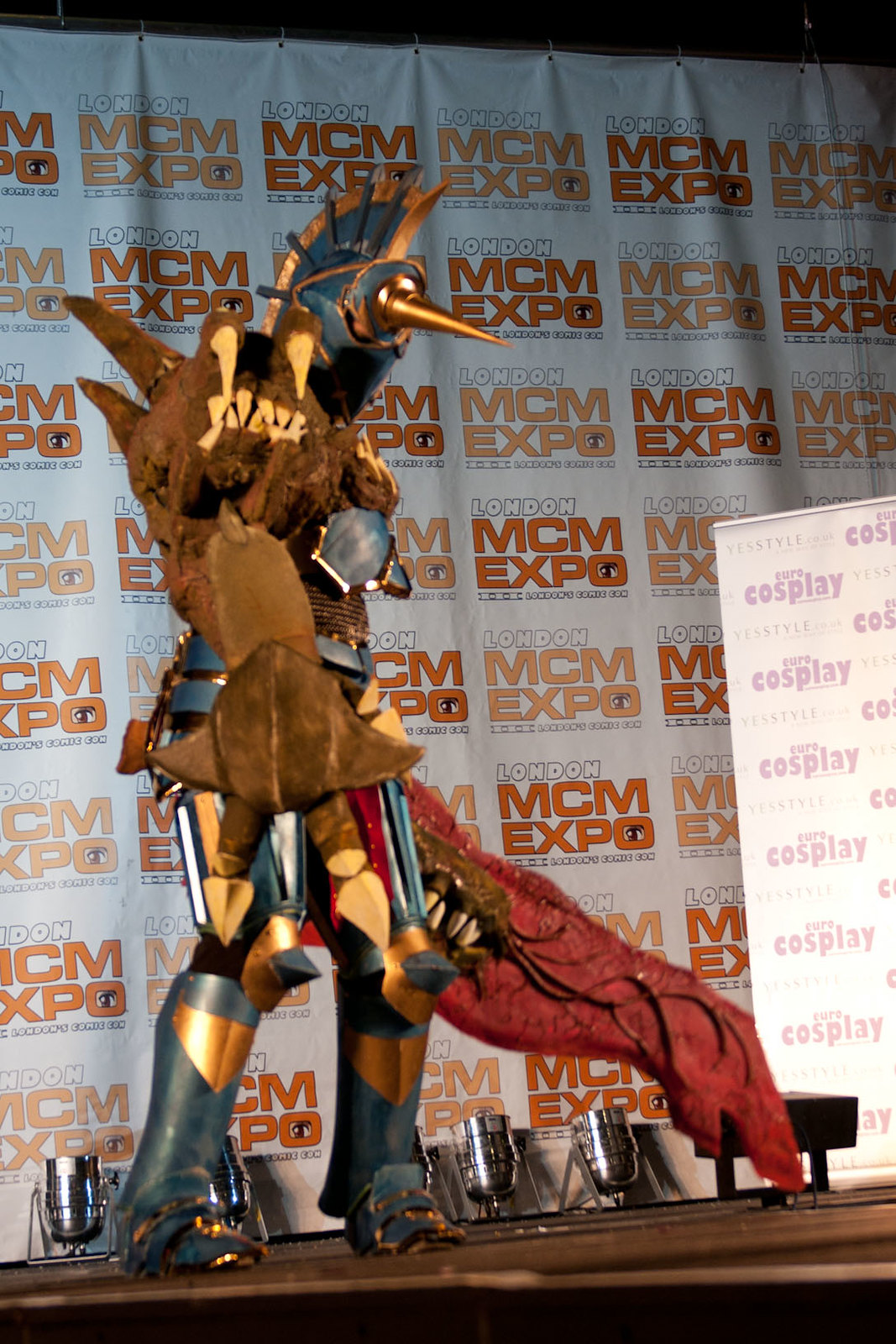This photograph captures an individual on stage at the London MCM Expo, participating in a cosplay event. The person is fully dressed in an elaborate suit of armor, characteristic of a knight yet with fantastical elements suggesting a fictional character. The armor is predominantly dark blue with intricate gold embellishments. A prominent golden unicorn horn adorns their helmet, which also features a fin extending from the back of the head to the neck. One arm is fitted with an oversized, claw-like appendage resembling a monstrous hand, and the other hand grips an extraordinarily large red sword designed to look like flesh. Visible behind the cosplayer are banners reading "London MCM Expo," along with additional references to "Euro Cosplay" and "Yes Style," signifying the event's location in London, England, and its themes of comic and cosplay culture.